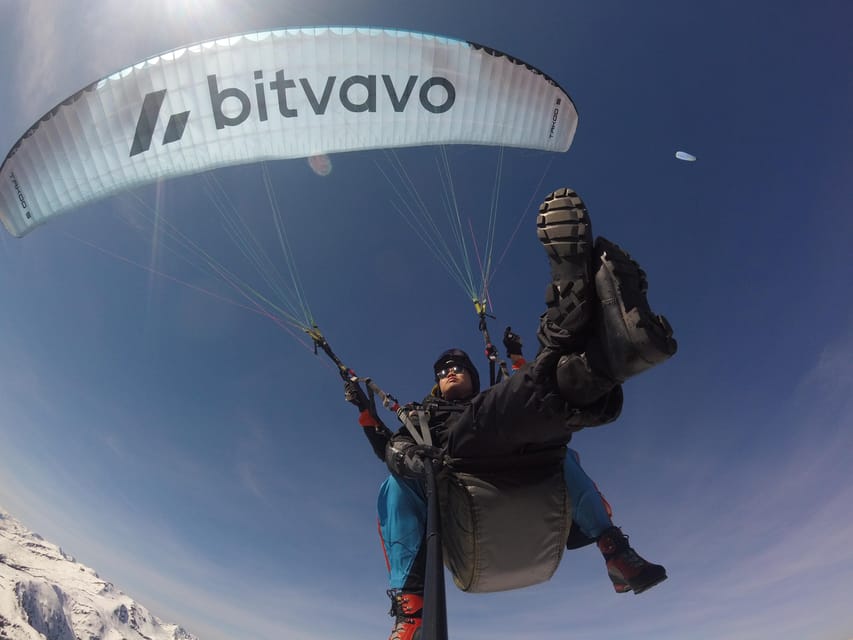This photograph captures a thrilling scene of two individuals engaged in tandem paragliding against the backdrop of a pristine, snow-covered mountain range. The paragliders dominate the frame, viewed from a vantage point that suggests the use of a selfie stick, allowing a wide, encompassing shot. The sky transitions from a deep indigo in the top right to lighter hues towards the earth, accentuating the clear, sunny conditions with a visible, brightening sun and minimal clouds. 

The parachute above them is predominantly white with black and blue accents, bearing the logo and the word "BITVAVO." The pilot, situated in the rear, is distinguished by a turquoise jumpsuit, orange snowsuit elements, and black boots. Only his legs are visible, confirming his controlling position. His passenger, ensconced in a pouch-like seat between the pilot's legs, is dressed in a black snowsuit, black boots with prominent tread, and sunglasses, suggesting bright, cold conditions. The passenger's relaxed posture, with legs stretched out and feet crossed, indicates a smooth glide, contributing to the overall serene and adventurous ambience of the photograph.